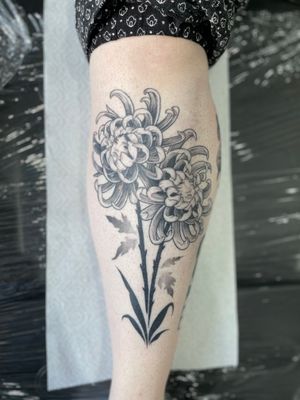The image features a detailed tattoo in black and white ink on the front of someone’s lower leg, positioned between their calf and knee. The tattoo is of two large flowers with intricate petals that converge at the base into long, slender stems and thin leaves. The centerpiece of the tattoo includes a woman's face within one of the petals. The leg, which appears to have white, Caucasian-looking skin, is clothed in pants with a rolled-up sleeve end, revealing the tattoo. The leg rests on a white, sterilized pad that sits atop a wooden table marred with white splotches. The background suggests a gray, possibly plastic-covered surface, adding to the sterile, clinical setting of the image.